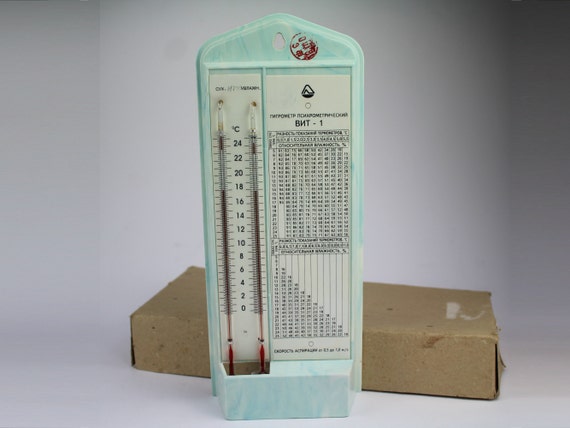The photograph depicts an antique device resembling a thermometer, standing upright. The left side of the device features two vertical mercury thermometers, each marked with a scale in degrees Celsius ranging from 0 to 24. In between the thermometers, the numbers are prominently labeled. Adjacent to the thermometers on the right, there are two charts filled with numerical data and text, which appear to be in a foreign language, making their exact purpose unclear but suggesting a reference tool akin to a multiplication table. The device has a light blue rectangular panel with a hole at the top, possibly for hanging or mounting. A clear tube, containing a reddish liquid, runs vertically along one side, indicative of a traditional thermometer's mercury design. The background reveals a worn and tattered cardboard box that appears to have originally housed the device, adding a sense of age and usage, and the overall color scheme and condition of the background is grayscale and heavily worn.